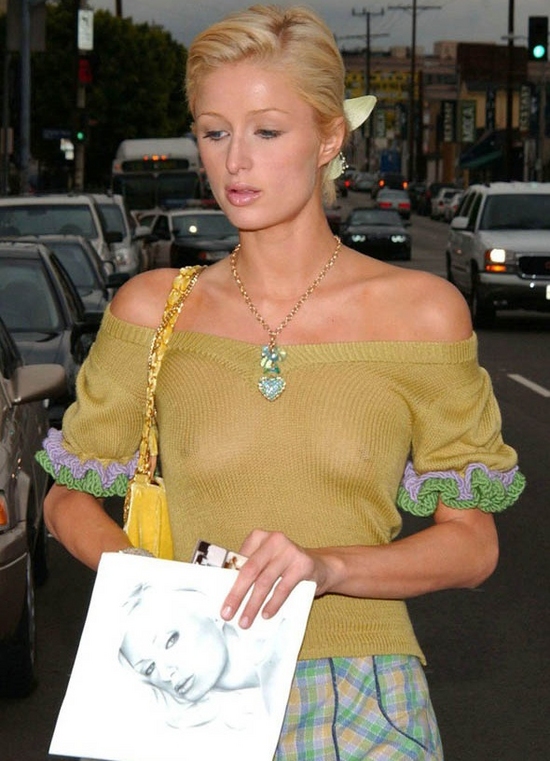Paris Hilton is captured standing on a bustling street, embodying a unique blend of glamour and casual style. She is wearing a yellow, sheer off-shoulder top that subtly reveals her shoulders and partially showcases her nipples beneath the fabric. The top is adorned with puffy, darker green and light purple sleeves that add a touch of playfulness to her outfit. Complementing this, she wears a green plaid skirt or pants. Her accessories include a yellow handbag, a delicate necklace with a golden chain and a green pendant featuring a bow and a heart, and a barely visible bracelet.

Paris's blonde hair is styled into a neat updo, possibly a bun or short ponytail, with a ribbon or bow peeking out from behind her head. In her right hand, she holds a black-and-white sketch of herself, with possibly another photo behind it. The background features an ordinary street scene with parked cars to her left and moving traffic to her right, along with buildings, street signs, power lines, and traffic lights, suggesting a typical urban environment at dusk.